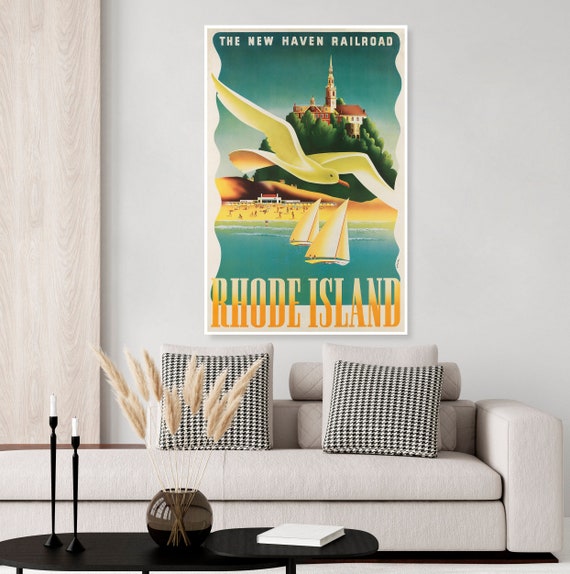The computer-generated image portrays a sophisticated living area, appearing as though it belongs in a high-end design magazine or decor advertisement. Central to the composition is a beige sofa adorned with an array of pillows: two white square cushions at the front, with two black-and-white checkered pillows positioned directly in front of them, and two grey cushions at the back. A sleek, modern black coffee table is placed in front of the sofa, featuring a dual-circle design—a larger circle and a smaller one. Atop this table are two tall black candleholders with white candles, a notebook, and a distinctive brown jar filled with approximately eleven white feather-like plumes. Suspended above the couch is a vibrant poster highlighting the New Haven Railroad of Rhode Island, featuring detailed illustrations of a seagull in flight, a small castle on a hill, sailboats, and people enjoying the beach. White walls and a white curtain to the left accentuate the bright and airy ambiance of the room, making the stylish elements of the decor stand out.